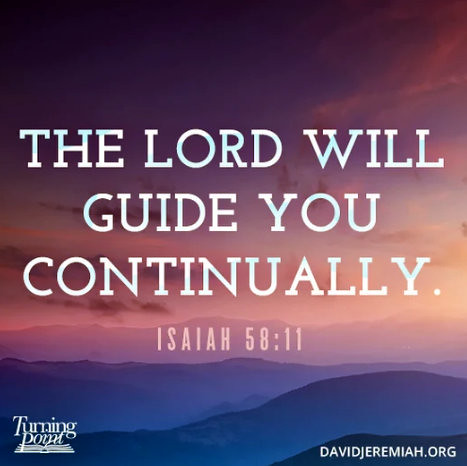The image is a square graphic featuring a religious quote from the Bible, prominently displayed in the center in large, capitalized white text that reads "THE LORD WILL GUIDE YOU CONTINUALLY" with "ISAIAH 58:11" also in all caps. The wording is aligned centrally, creating a focal point. The quote is attributed to davidjeremiah.org, which is printed in the lower right corner, while "Turning Point" is marked on the lower left corner. The background image is a striking scene that looks heavenly, depicting a landscape with a dark upper sky transitioning to a lighter pink towards the horizon. Below the sky lies a mountain range, rendered in black with white mist rising up, suggesting either dawn or dusk. The overall impression is serene and inspiring, creating a perfect backdrop for the uplifting message.